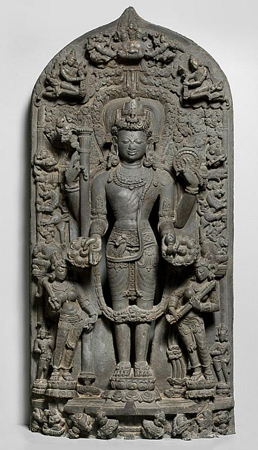This image depicts an intricate, dark gray stone carving resembling an ancient Egyptian artifact, possibly from a museum collection. The carving is tombstone-shaped, with a pointed arch at the top and 90-degree angles at the base. Centered on the stone is a detailed figure of a woman with closed eyes, an Egyptian headdress, and a robe tied with a rope belt. Surrounding her are smaller figures: two women standing to her right and left and another tiny figure to the left. These figures appear to be holding something indistinct. Additionally, there may be depictions of snakes and other complex carvings embedded into the stone's designs, with even more figures etched into the top of the piece. The entire carving appears against a cream-colored background, enhancing its ancient and mystical aura.